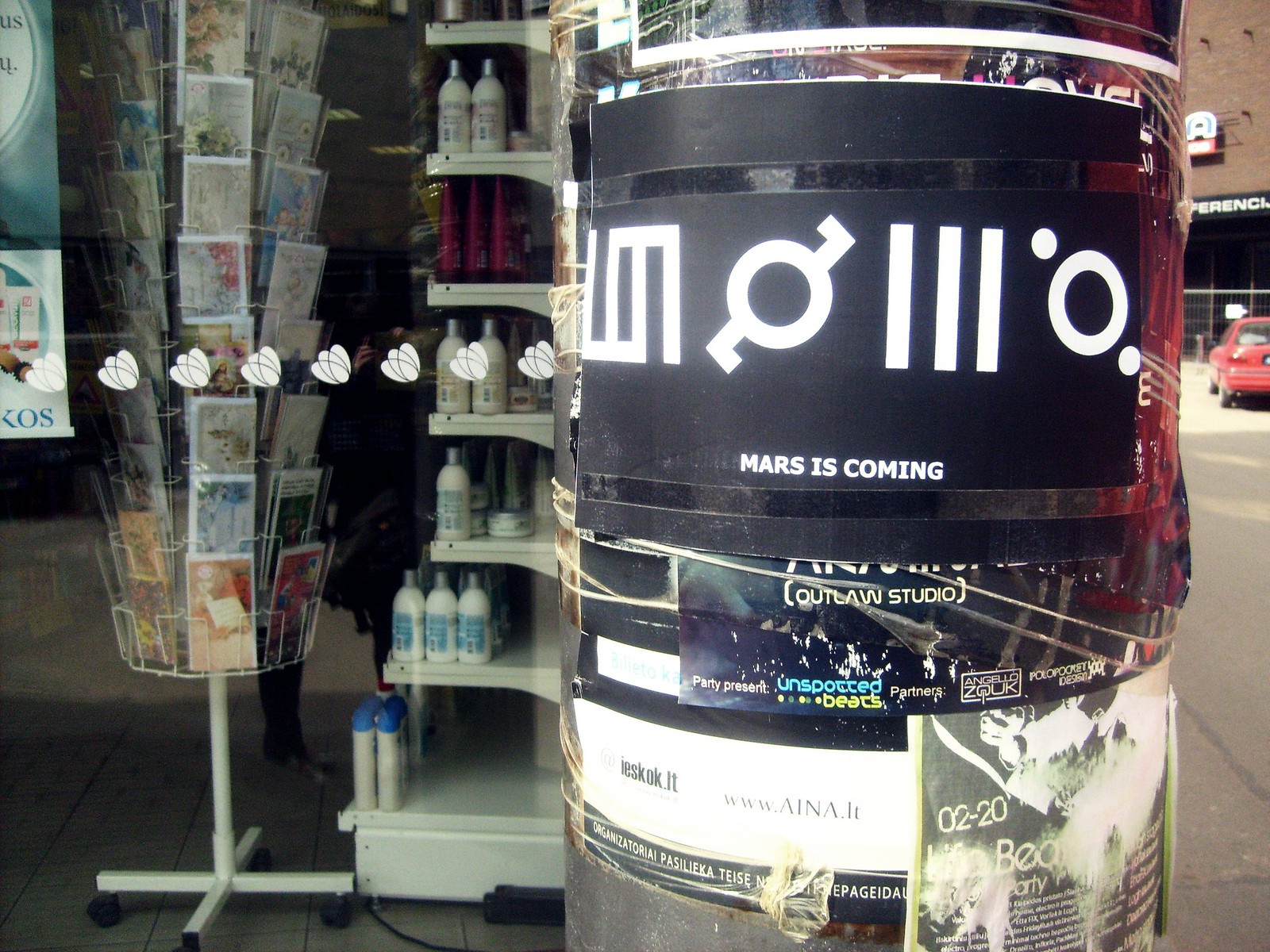The image captures a vibrant street scene. On the left side, there's a store window displaying an eclectic array of postcards and greeting cards in a white rack, featuring an array of colors like blue, red, gold, brown, beige, pink, and green. Right next to the postcards, there are several white shelves stocked with various beauty and hygiene products. Each shelf holds bottles meticulously organized by color and type: the top row is lined with white bottles capped with silver lids; below that, rows of purple bottles with black lids and more white bottles with alternating silver and blue lids are arranged. Overhead, against the far left top corner, "KOS" in blue text stands out on a white background, while a white circular logo with blue text contrasts against a gray backdrop. The floor appears tiled in gray.

On the right side of the image stands a street post plastered with numerous flyers and posters; the most prominent is a black poster with unusual symbols above the white text that reads "Mars is Coming." A background of a reddish-brown brick building partially obscures a silver gate and a red car parked across the gray street, marked by yellow lines in the middle. The overall scene exudes a bustling urban atmosphere with a mix of commercial and street elements.